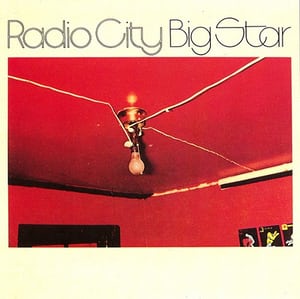The image features a small, square photograph set against a pastel yellow background. At the very top, in thin black letters, the text reads "Radio City Big Star." Below the text is a photograph primarily showcasing the ceiling and far corner of a room, both painted in a vivid red. The centerpiece of the ceiling is a gold light fixture, which lacks a shade and houses a single light bulb with a pull chain. The ceiling is marred by three distinct white cracks: one extending to the left and two branching off to the right. Additionally, there are white wires stapled to the ceiling, extending from the left, top right, and far wall, all converging at the light fixture. On the wall, though partially visible and indistinct, some pictures or posters are hanging. The photograph gives the impression of an album cover with its meticulous details and emphasis on the ambiance created by the sparse yet stark elements.